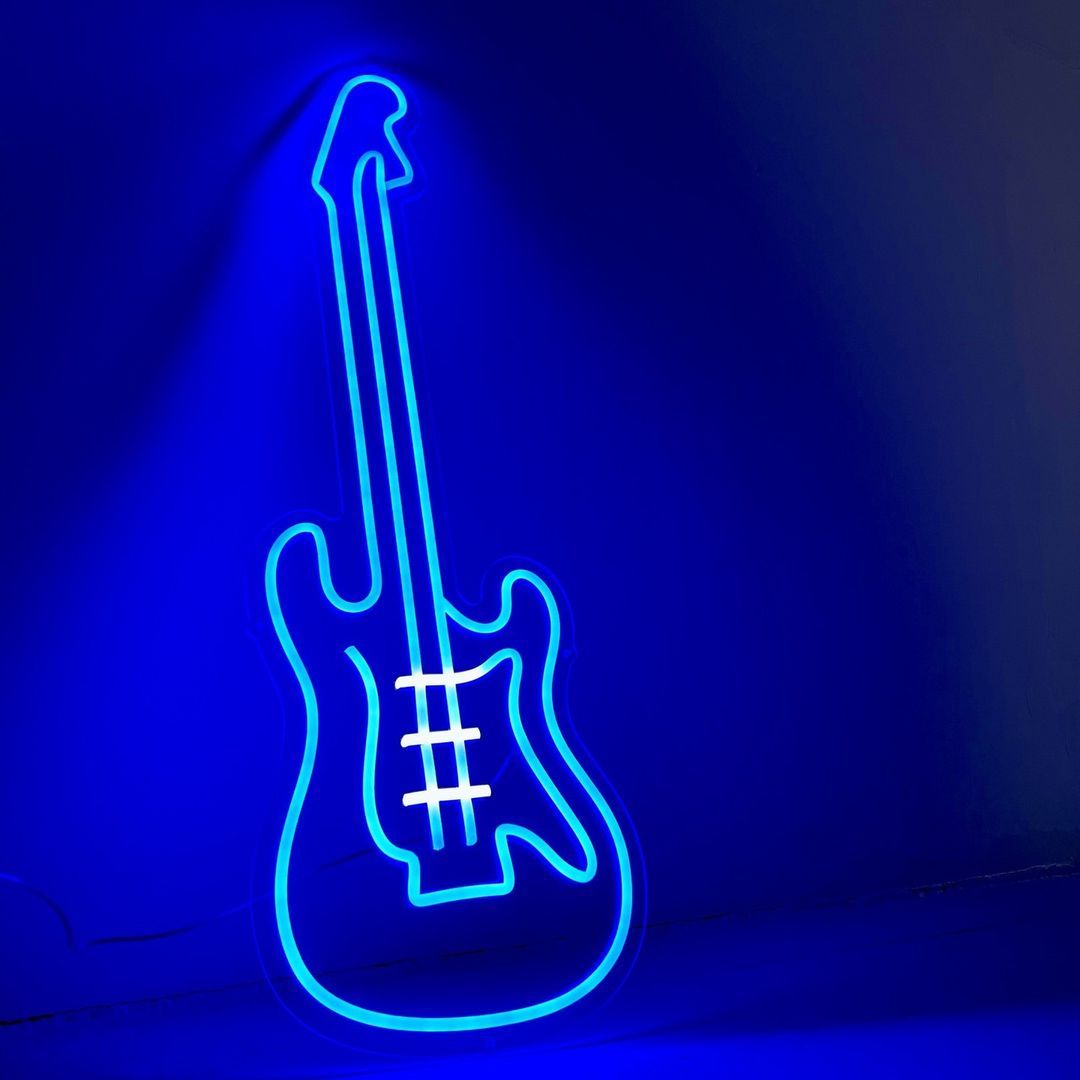The image showcases a detailed and high-quality LED neon light-up of an electric guitar, primarily in shades of turquoise and electric blue, with white neon strings. Positioned against an electric blue background, the guitar has an iconic shape with two horn-like structures at its base flanking the neck. The neon artwork employs a single continuous piece for the guitar's outline, while separate neon pieces add interior definition. Three distinctive white lines represent the guitar strings toward the bottom. The background, while fainter and darker, accentuates the luminous quality of the guitar, lending the entire composition a vibrant and striking appearance. No additional objects or text clutter the image, ensuring full focus remains on the brilliantly lit, intricate design of the guitar.